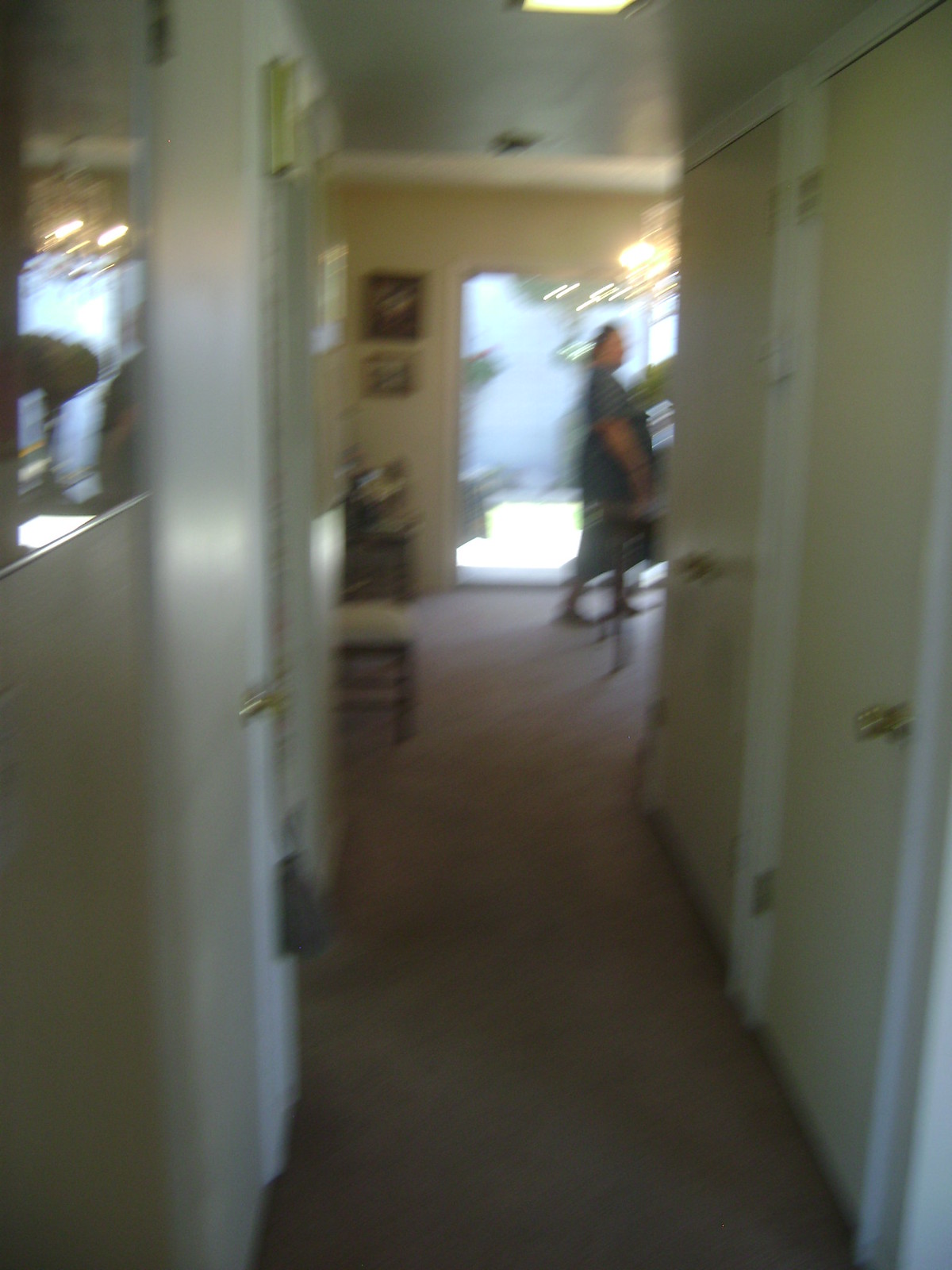This slightly out-of-focus photograph captures a domestic interior scene from the perspective of the end of a hallway leading into a living room. The hallway features two closed doors, one on each side, both adorned with gold doorknobs. The image incorporates a glimpse of the living room beyond, where a woman dressed in a short-sleeved blue shirt that extends past her hips and some kind of pants is seen walking across the floor. Behind her, large sliding glass doors allow natural light to fill the space. To the left of these sliding doors, two pictures hang vertically on the wall, with a larger one positioned above a smaller one. Additionally, a wooden chair is visible at the left-middle section of the image, adding to the cozy, lived-in feel of the room.